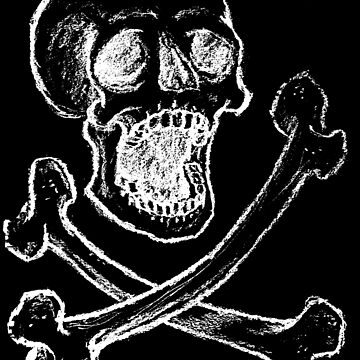This illustration features a chalk-style drawing of a skull and crossbones on a solid black background. The skull, depicted in white chalk, is oriented towards the right with a slight tilt, revealing wide eye sockets and a gaping mouth suggestive of a scream. The detailed eyes and mouth are fully colored, adding depth to the expression. Beneath the skull are two crossed bones, drawn with an organic, curved form rather than straight lines. The longer bone extends from the top right corner to the bottom left, notably arching outward, while the shorter bone spans from the bottom right to the top left, showing a gentler curve. The entire composition is rendered in a way that emphasizes the textured, drawn appearance of white chalk on a black background. The skull prominently displays its skeletal teeth, enhancing the eerie, expressive nature of the image.